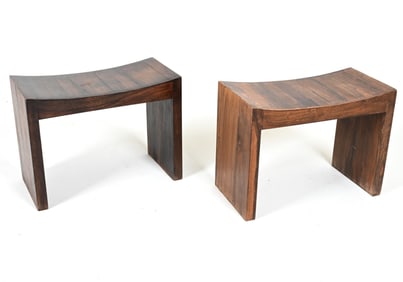The image features two wooden benches set against a plain white background with subtle shadowing beneath them. The bench on the left, positioned slightly further back, is crafted from a darker wood, while the bench on the right, placed a bit more forward, is made from a lighter wood. Both benches exhibit a unique design with an indented top that curves inward, creating a dip in the middle. Instead of traditional legs, each bench features two wide wooden slabs on either side, seamlessly grounding them to the floor. The design elements and placement on the stark white background emphasize the simplicity and craftsmanship of the benches without any additional context.